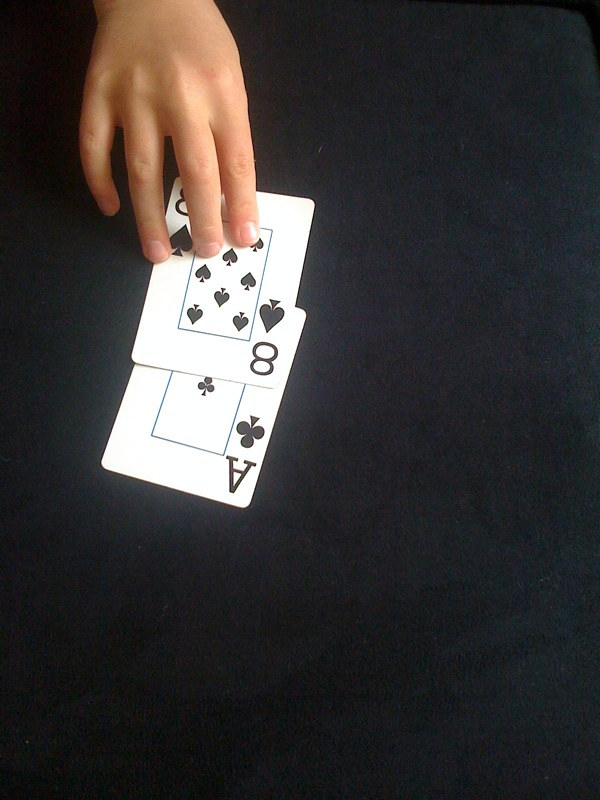A detailed color photograph in portrait orientation captures the moment of a child playing cards on a dark, featureless table. The small right hand, with short fingernails, is prominently featured at the top of the image. The thumb is not visible as it extends from the top part of the frame downwards. The forefinger, middle finger, and ring finger are resting on an Eight of Spades card, which is placed atop an Ace of Clubs. Shadows, likely cast by the child and possibly another person outside the frame, add depth to the scene, with noticeable darker areas at both the top and the bottom left of the photograph. The simplicity of the dark table surface contrasts with the vivid details of the playing cards and the child's delicate hand.